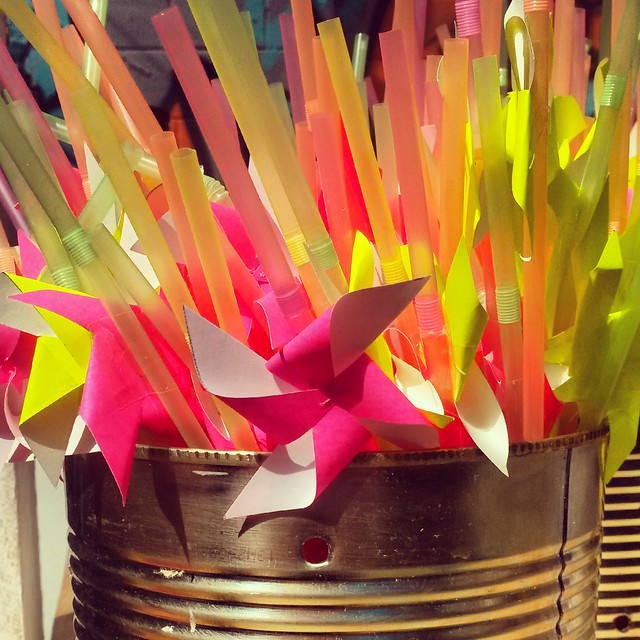This image showcases a festive decoration likely intended for a summer party, possibly for a little girl. Positioned on a flat surface, the main feature is a silver, ridged metal can or bucket, which might have been a repurposed soup can with its label removed. This container is filled with an array of colorful, clear neon straws in hues of pink, yellow, green, and orange. Some of the straws have attached pink pinwheels or paper mache fan-like decorations in pink and yellow, adding to the vibrant and playful aesthetic. Intriguingly, there appears to be a second similar container visible behind the main one, contributing to the overall festive and cheerful ambience of the scene.